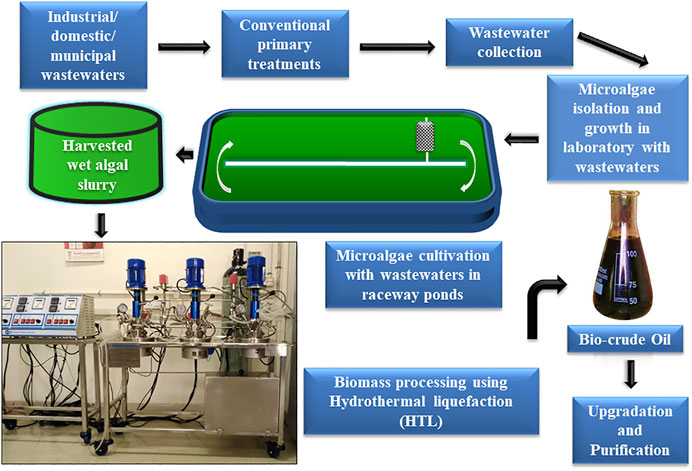The image features a detailed flowchart in green and blue block-style typography, complete with one photograph in the lower left corner. The photograph showcases a laboratory setting, equipped with several stainless steel trays and numerous buttons.

The flowchart begins with the input of industrial, domestic, and municipal wastewaters, which flow into conventional primary treatments. This leads to wastewater collection. Next, the diagram moves to the microalgae isolation and growth phase within a laboratory setting using these wastewaters. The growth process is visually represented by an image of isolated algae in a rectangular tank. 

Following this, the flowchart depicts the harvesting of wet algae, which then transitions back to the laboratory environment. This is where the photographed setting with silver trays and buttons is placed, indicating the phases of processing. To the right of this, the chart details biomass processing through Hydrothermal Liquefaction (HTL), resulting in bio-crude oil. This stage includes an illustration of a testing bottle filled with a dark oil substance, complete with measurement markings.

Finally, the flowchart concludes with the stages of upgrading and purification of the produced bio-crude oil.